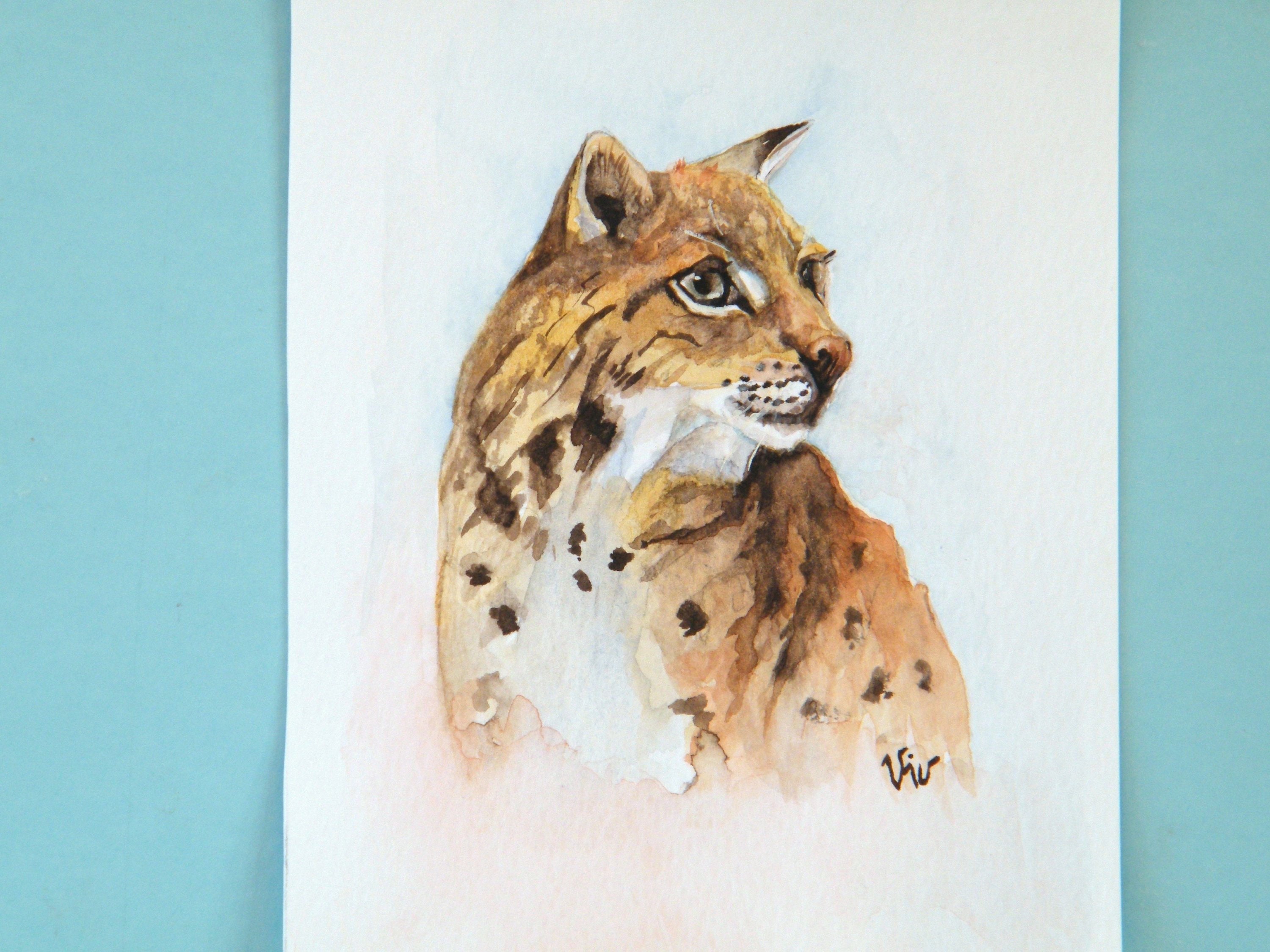The image depicts a traditional painting, likely crafted with watercolors or possibly oils, featuring a feline that resembles a bobcat, a small tiger, or another large cat species. The animal, with its pointy ears and yellowish-orange fur accented with brown and black spots, is posed with its body oriented to the left while its head is turned toward the right, giving it a dynamic and engaging appearance. The painting has blurred edges typical of watercolor and the ink bleeds into the paper, adding a textured and abstract feel to the body, while the face remains more detailed, highlighting features such as the spots around its mouth. The feline is depicted on a white piece of watercolor paper, which sits against a soft blue background that appears on either side of the paper. The bottom right corner of the painting features a signature, most likely "V.I.V" or "V.I.B," written in dark brown.